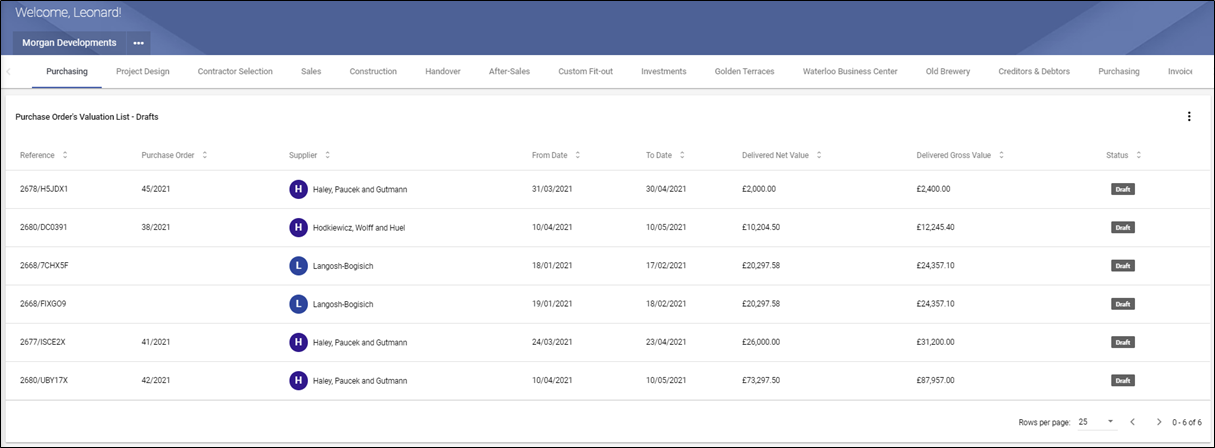The image is a screenshot of a personalized webpage for Leonard, prominently displaying "Welcome, Leonard" at the top. The website appears to belong to "Morgan Developments" and features a small logo against a blue-bordered background. Along the top navigation bar, "Purchasing" is underlined in blue, indicating the current active section. Below this, the page is organized into multiple columns, consisting of lists of items that are difficult to read in detail.

The first column contains approximately six text entries. The second column seems to display numerical values. The third column features blue circles, each containing a letter. In the fourth column, there are pairs of dates, indicating a range "from" and "to." The next columns include what appears to be prices, and the last column possibly lists the status of each entry, although the text is hard to discern. Each row is bordered by blue boxes, and the table extends down to the bottom of the page.

At the very bottom, pagination options are visible, allowing users to navigate through the pages by clicking left or right arrows.